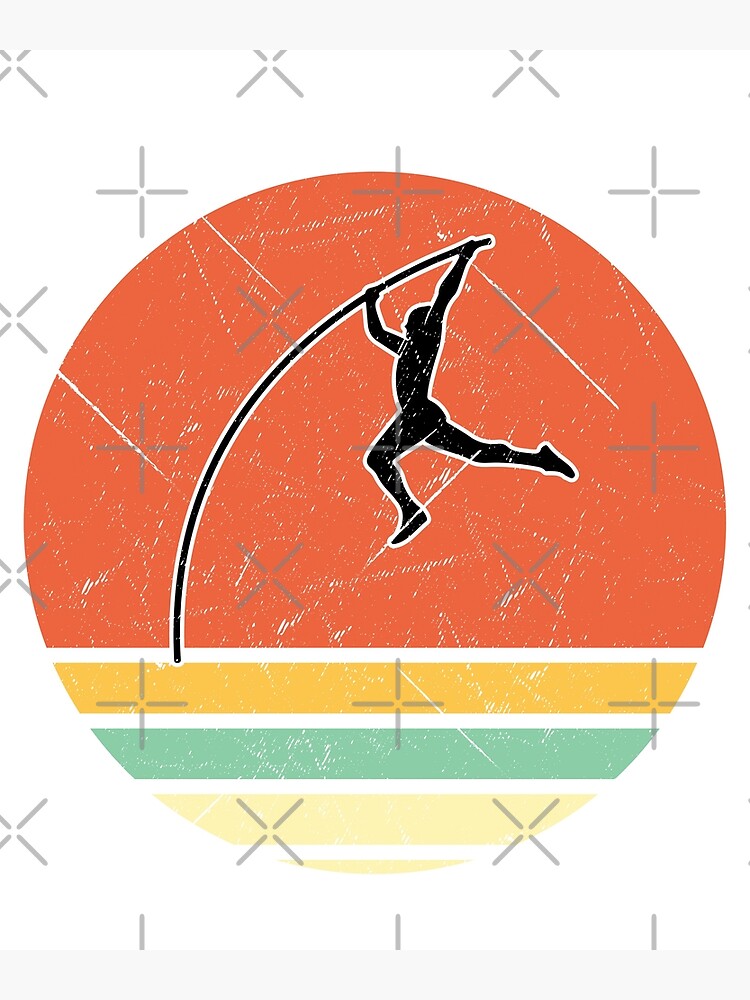The image showcases a detailed graphic design centered around a circular shape against a white background. At the core of the circle is a striking black silhouette of a pole-vaulter mid-leap, clutching a bent pole that forms an arc. The circular frame is divided into several color segments: the top two-thirds is filled with a vivid red, while the bottom features four horizontal stripes in yellow, green, pale yellow, and light yellow, separated by thin white lines. Surrounding this central illustration is a white border, providing a clear separation from the diverse background colors. The entire image background is white, adorned with gray, cross-shaped, and X-shaped symbols scattered throughout. Additionally, gray bars extend along the top and bottom edges of the image. The circle itself displays subtle textures, suggesting visual effects like scratches or light imperfections, enhancing the design's depth and visual interest.